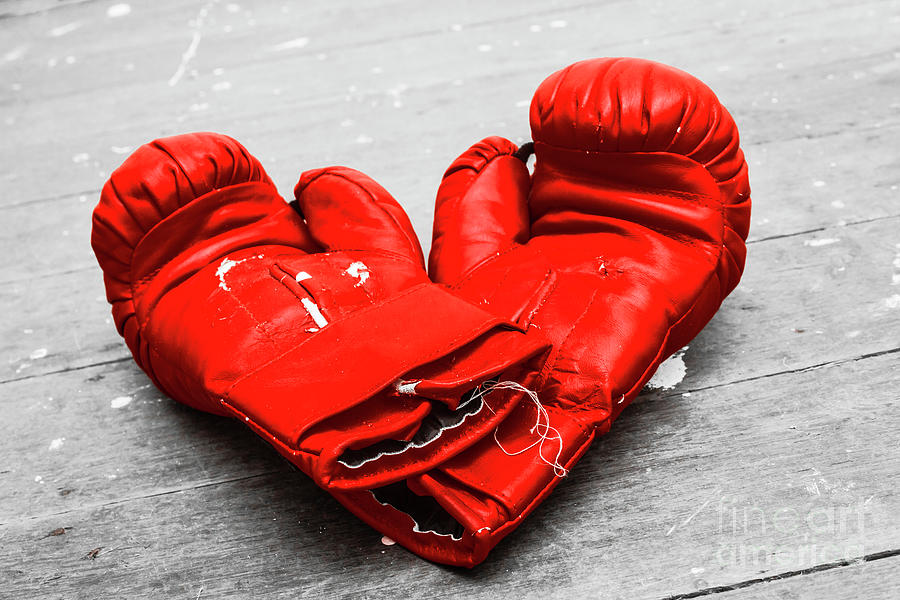This photograph captures a pair of significantly worn, fire engine red boxing gloves positioned palm side up on a severely weathered, grayish wooden floor. The gloves are slightly stacked with their wrist portions overlapping, forming a heart shape with the rounded finger ends sticking out to the left and right. The red leather fabric of the gloves is heavily stripped in areas, revealing the white underside, and there are dangling threads along the cuffs, emphasizing their age and usage. Subtle white splatters dot the worn wooden planks underneath, adding to the vintage, muted aesthetic. The image is watermarked with "Fine Art America" in the lower right-hand corner.